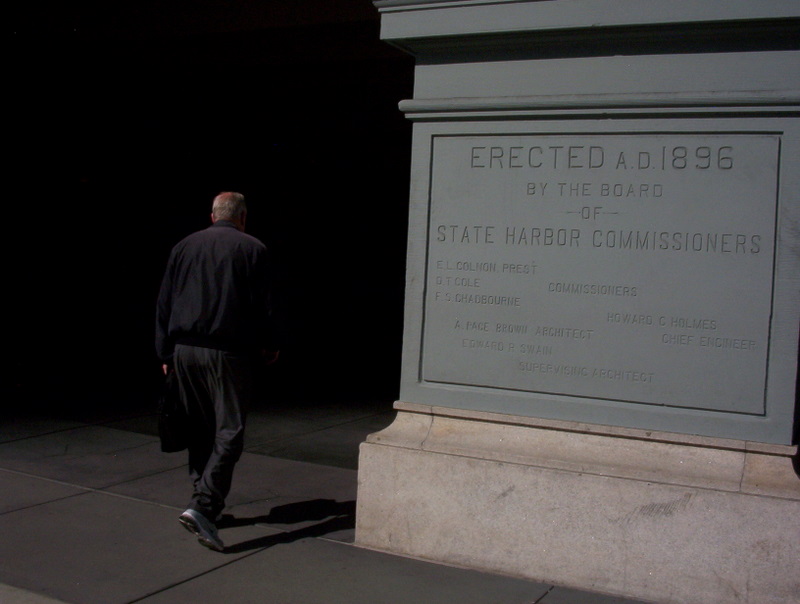In this nighttime scene, there's an imposing stone monument with a dull green hue, standing massive and solemn on a concrete foundation. The pillar, measuring approximately seven feet wide, bears inscriptions etched into its surface, reading "Erected A.D. 1896 by the Board of State Harbor Commissioners." Listed are names such as "E.L. Coleman Prest," "D.T. Cole," "F.S. Chadbourne," "P. Howard," "C. Combs, Chief Engineer," "Edward R. Swain, Supervising Architect," and "A. F. Brown, Architect." To the right of this brightly lit pillar, an elderly man with graying hair hurriedly walks away from the light. He is dressed in a navy sweatshirt, black tracksuit pants, and gray athletic shoes, carrying a bag in one hand. His figure casts a shadow on the stone path, adding to the scene's eerie ambiance as he heads into a much darker, almost ominous area.